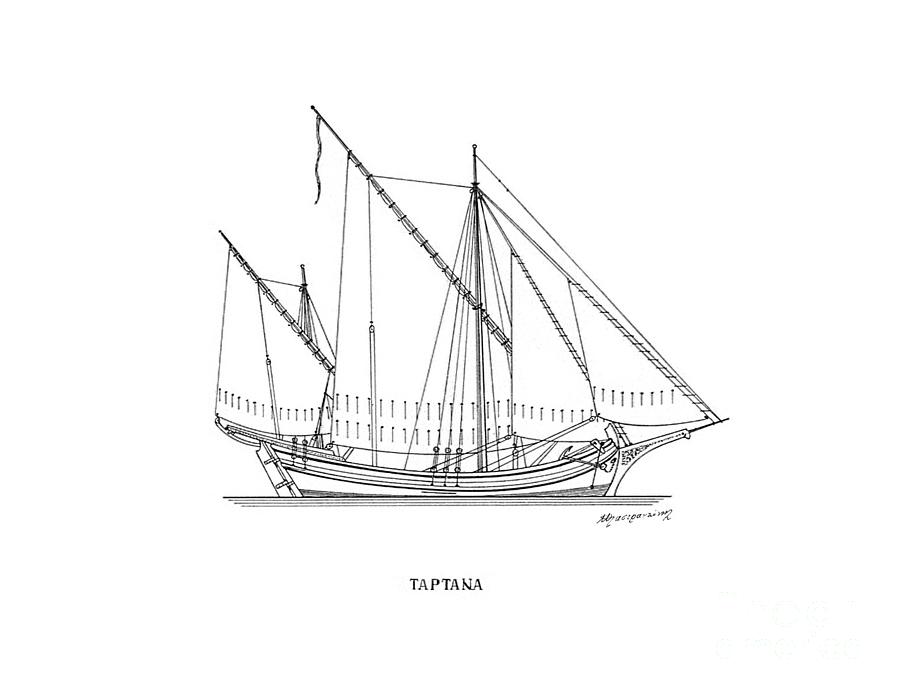This black and white sketch depicts a boat, elegantly stationed at a pier. The boat, seemingly wooden, showcases a classic design with four prominent sails catching an imagined breeze. Below the boat, text inscribed reads "TAPTANA" in clear, uppercase letters. In the lower right-hand corner, another text, written in cursive and appearing less legible, adds an air of authenticity to the artwork. The meticulous detail in the sails and the overall structure of the boat highlights the craftsmanship and artistry involved in this sketch.